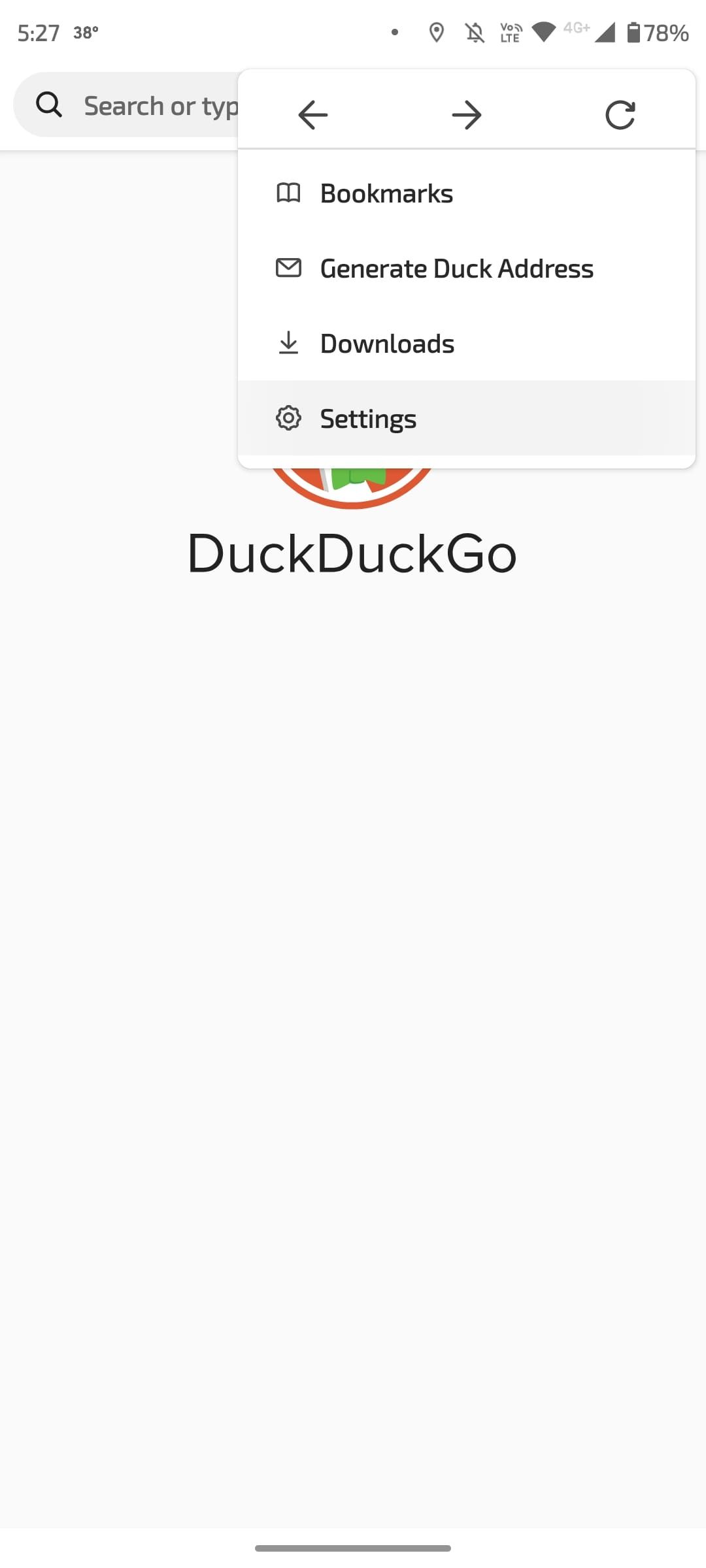This grayscale image appears to depict a screenshot of a mobile device's browser interface. In the upper portion, black font displays the time as 5:27 and the temperature as 38 degrees Fahrenheit. Adjacent to this, on the right, a series of icons line up: a black dot with a GPS logo, a no notifications icon, a VOLTE icon, a Wi-Fi signal icon, a 4G+ symbol, and a battery life indicator showing 78% remaining.

Directly beneath these status icons is a search bar featuring a magnifying glass icon and the text "Search or type." To the right of the search bar are navigation buttons including back, forward, and refresh. Additional options like bookmarks, generate duck address, downloads, and settings are also visible.

Centrally positioned in the image is the DuckDuckGo logo, characterized by an orange circular background with a duck donning a green bowtie in the center. The overall appearance suggests a user interface centered on functionality, with the DuckDuckGo search engine as the focal point.